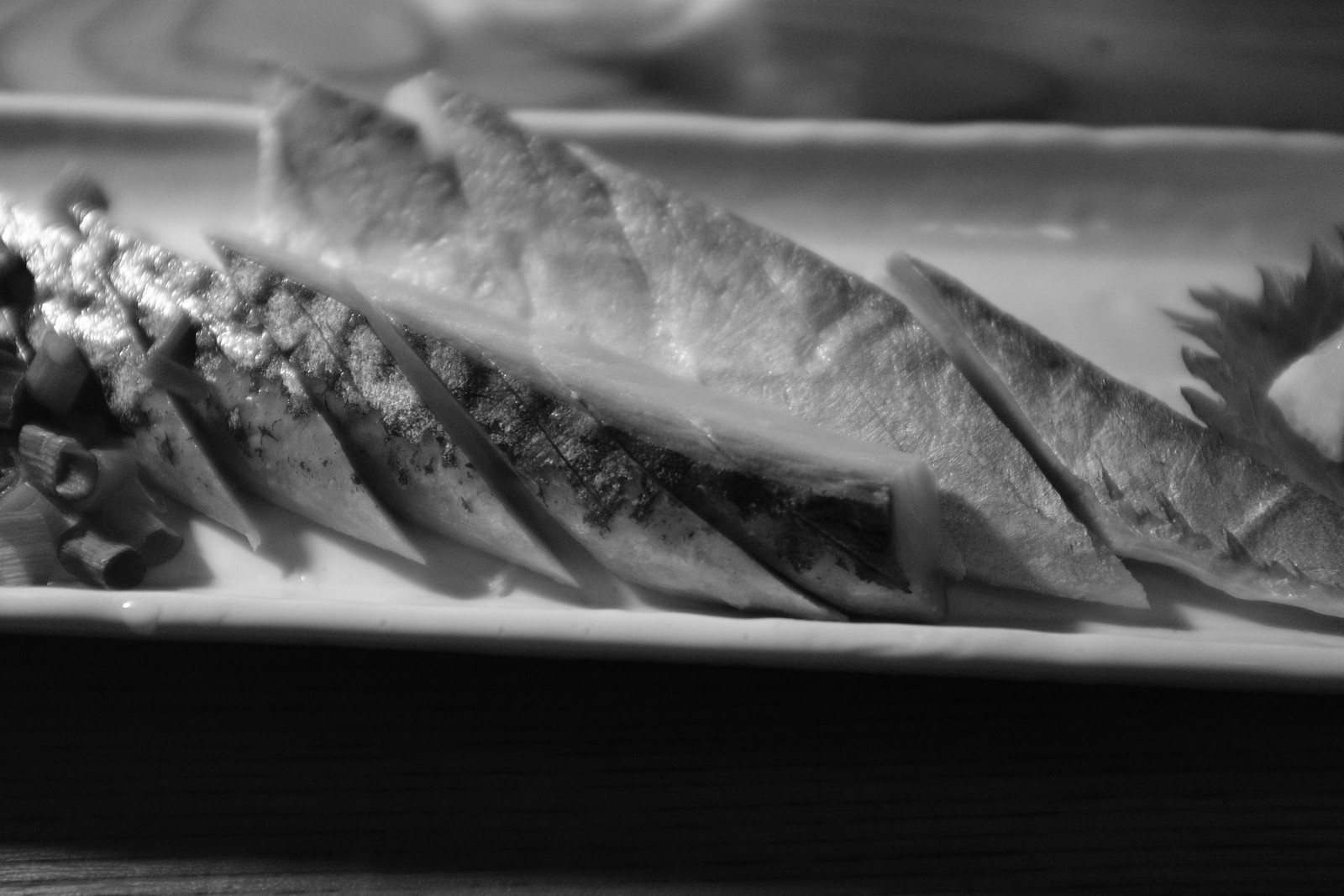In this black and white photograph, a sleek, elongated tray is prominently positioned at the center, stretching horizontally from left to right. The tray resembles a sliced pipe, forming a cupped half-cylinder shape that cradles an ambiguous food item. The item appears sliced and exhibits a smooth surface that could either resemble the texture of fish skin or a glossy pastry exterior. The background is predominantly black, with a blurred upper portion, likely suggesting an indoor setting, potentially at a fancy restaurant. The image contains no text, focusing entirely on the visual elements of the tray and the mysterious food it holds.